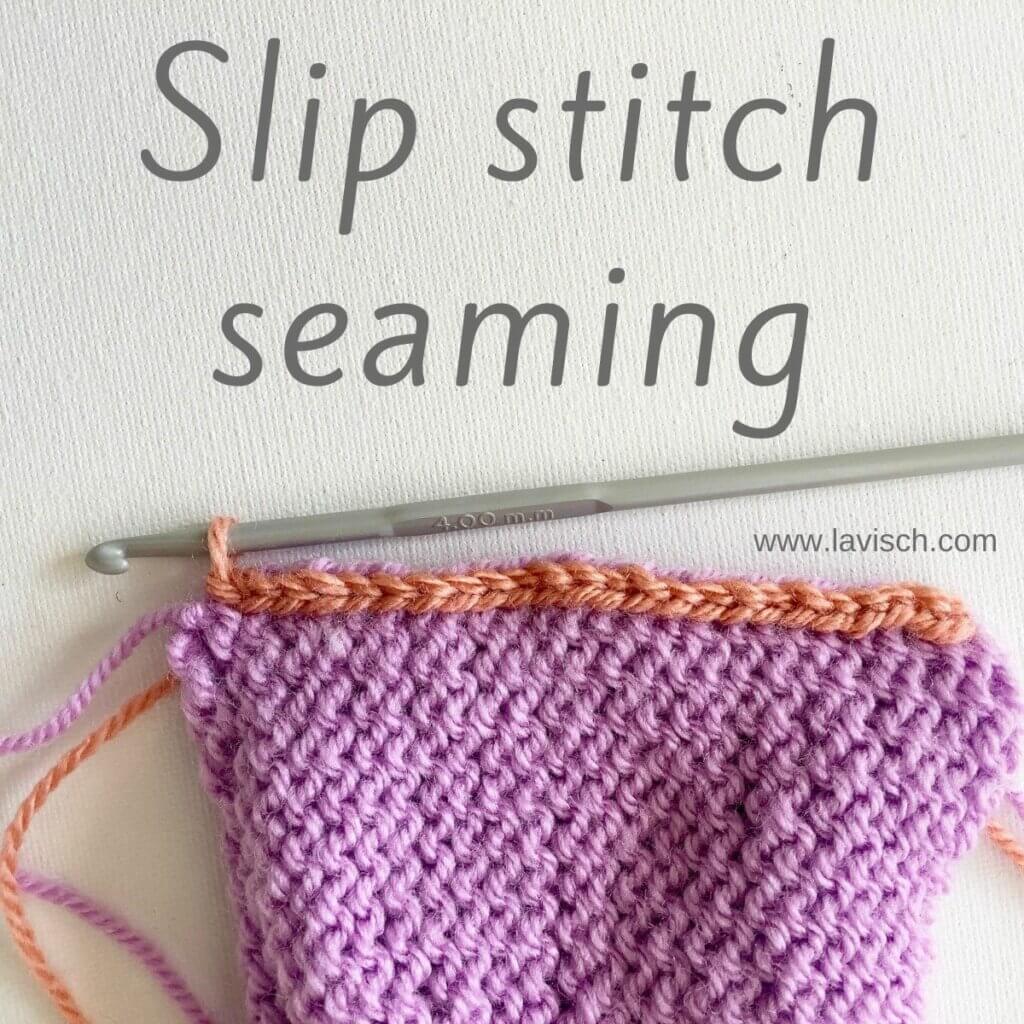This detailed photograph showcases a crocheted project that is currently in progress, lying on a white or off-white cloth background. The focal point includes a gray crochet hook labeled "400mm," positioned in the middle of the scene. The project features two types of yarn: a majority of it is light purple or lavender, while the upper border is made with a darker, rust-colored orange yarn. Text across the top of the image reads "Slip Stitch Seaming" in large, thin, gray letters, indicating the technique being used. At the bottom of the photo, just beneath the crochet hook, the website "www.lavish.com" (spelled L-A-V-I-S-C-H) is clearly visible. The project appears to involve teaching or demonstrating a DIY crochet technique, with emphasis on the slip stitch seaming method.